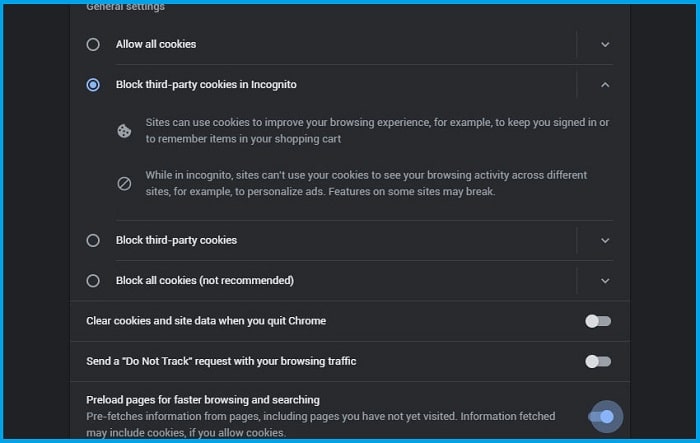The image shows a digital settings menu with a black background, lined and bordered in blue. At the top left, there's an unselected option labeled "Allow all cookies," alongside a dropdown arrow on the right. Below, a selected option reads "Block third-party cookies in Incognito," indicated by a solid blue dot inside a circle, with an upward-pointing arrow on the right.

An indented section below this provides further information: "Sites can use cookies to improve your browsing experience. For example, to keep you signed in or to remember items in your shopping cart." This section is accompanied by a cookie icon with a bite taken out of it.

Further down, an icon of a circle with a slash through it introduces more details: "While in Incognito, sites can't use your cookies to see your browsing activity across different sites, for example, to personalize ads. Features on some sites may break."

Other unselected choices in white text include "Block third-party cookies" and "Block all cookies (not recommended)." Two additional options, marked as turned on, are "Clear cookies and site data when you close Chrome" and "Send a 'Do Not Track' request with your browsing traffic."

Finally, there is an option labeled "Preload pages for faster browsing and searching," explained as pre-fetching information from pages, including those not yet visited. This option includes a note that fetched data may include cookies if cookies are allowed, and it is indicated as turned on by a blue dot.